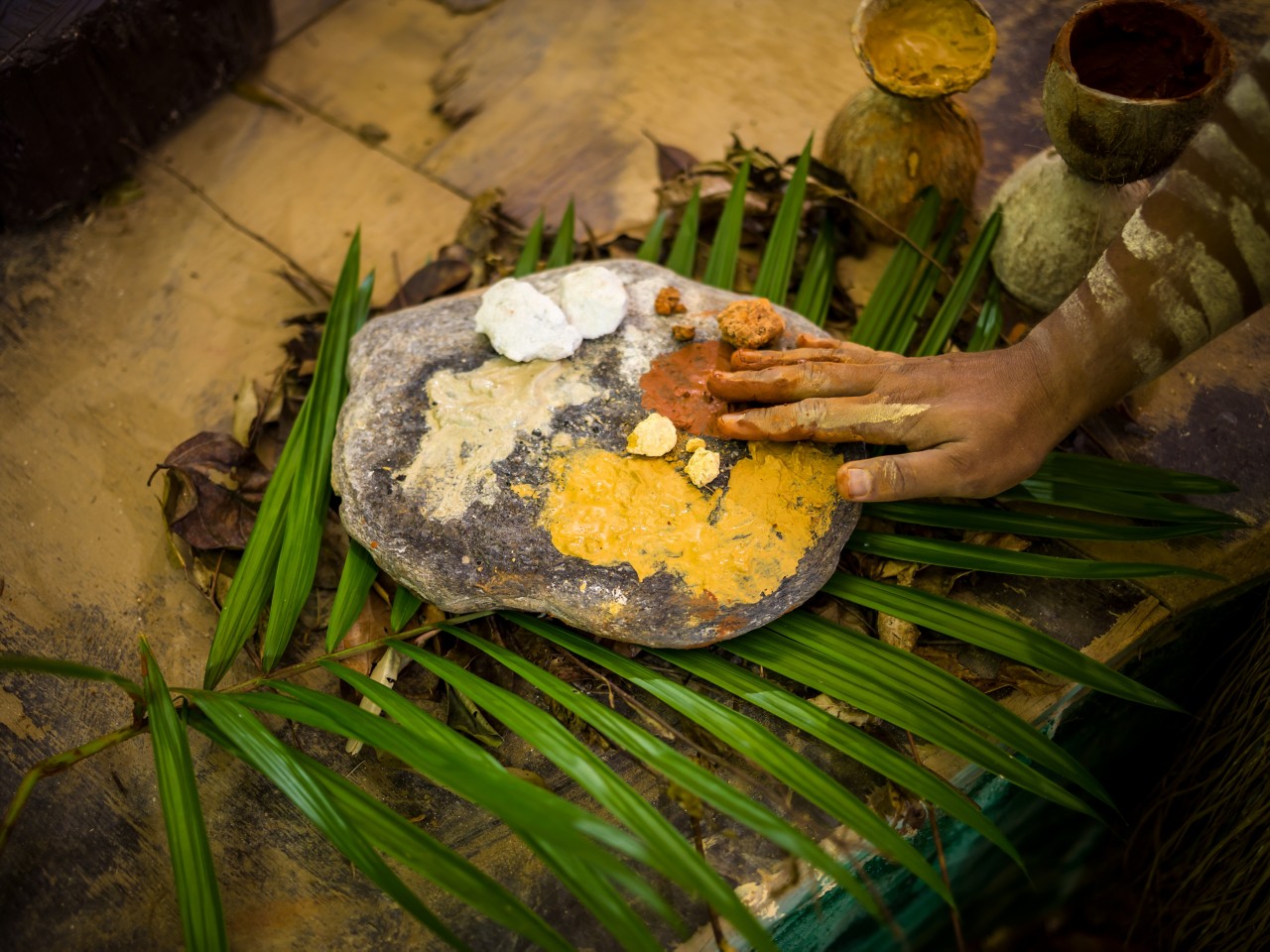An image captures a close-up scene where a person is mixing powdered paints or dyes. Their slightly dark-skinned hand, adorned with splotches of yellow and orange paint, extends from the right side of the frame, fingertips touching a circular, stone dish. The dish, resting atop a large palm leaf, holds an array of vividly colored powders — yellow, beige, white, orange, and brown-red. The palm leaf itself lies amidst darker green foliage, set on a table crafted from palm husk or palm wood, distinguishable by its teal-colored edge. Two coconut chalices, also splattered with yellow and orange paint, are positioned to the upper right of the image, adding to the scene's vibrant, tropical atmosphere. None of the paints in the tray have been mixed yet, suggesting a moment of artistic preparation.